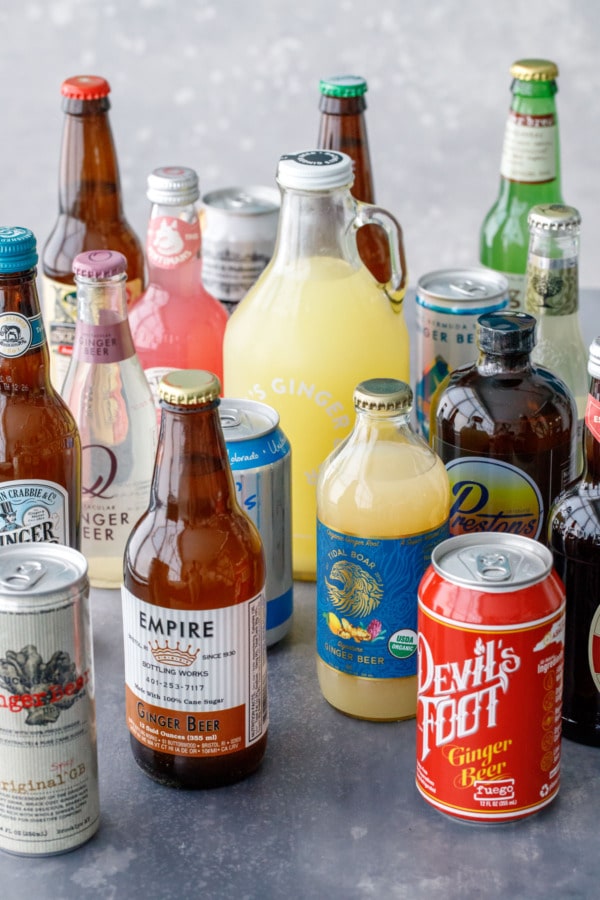The image depicts an array of 17 different varieties of ginger beer, meticulously arranged on a flat surface. Dominating the foreground is a vibrant red can of Devil's Foot Ginger Beer labeled "Fuego," indicating a spicy variant. Adjacent to it is a brown bottle of Empire Ginger Beer with a brass-colored cap. To the left of these, a clear bottle with a blue label reads "Large Ginger Beer." The collection features an eclectic mix of bottles and cans in diverse colors and shapes, including pink, green, and clear bottles, along with various cap colors such as silver, blue, green, and gold.

The backdrop consists of an all-white upper section transitioning into a blue and white lower section. Noteworthy amongst the bottles are a clear bottle with pink liquid and a silver cap, a brown bottle with a blue cap, and another clear bottle with a purple label partially covered yet legibly marked with "Ginger Beer." A striking detail is a bottle with yellow liquid and a white cap labeled with "Ginger" on a white background, placed centrally. Surrounding this are cans and bottles with labels featuring a mix of colors such as white, gray, black, blue, and gold.

Also highlighted in the image is a slender, tall aluminum can on the left and another distinctive bottle labeled Preston's in blue on a white and yellow background, contained in a dark brown bottle with a matching blue cap. Additionally, a bottle bearing a red cap and another with a green cap are positioned in the background, alongside various other bottles and cans each sporting unique labels and designs, contributing to a vibrant and diverse showcase of ginger beers.